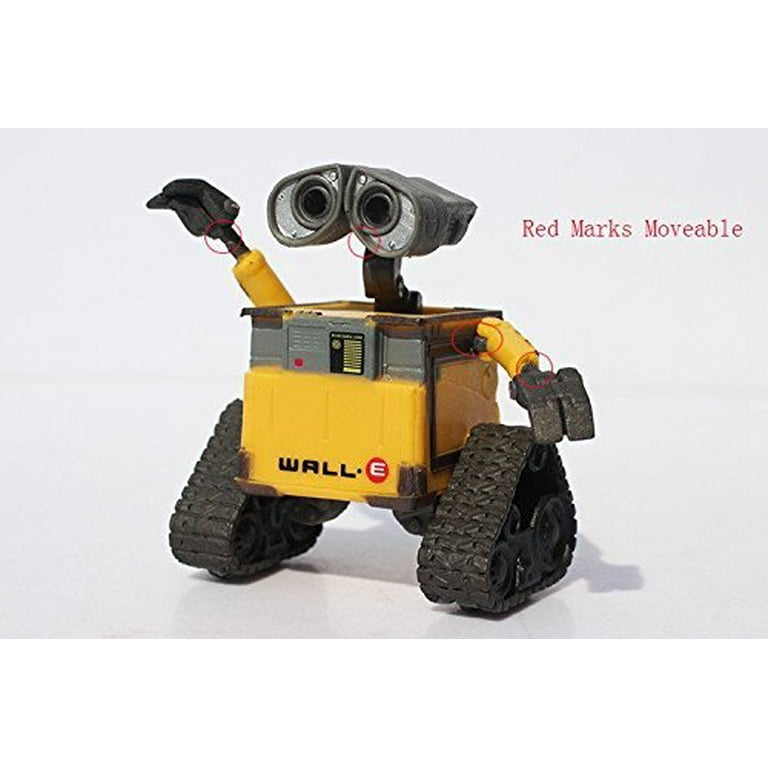This image features Wall-E, the endearing robot from Disney-Pixar's Wall-E movie. Wall-E has a bright yellow, square-shaped body with reinforced corners and a gray control panel band at the top. The front of his body prominently displays his name, "WALL-E," in black and white lettering. His head resembles a pair of binoculars, giving him expressive eyes. Wall-E's arms, equipped with claw-like hands that can articulate in different directions, extend from the sides of his body. Notably, red circles highlight movable joints around his neck, wrists, and one shoulder, indicating parts that are designed to move. His mobility is facilitated by two triangular treads, resembling tank tracks, that propels him forward. This scene is set against a clean white background, emphasizing the robot's detailed and functional design elements.